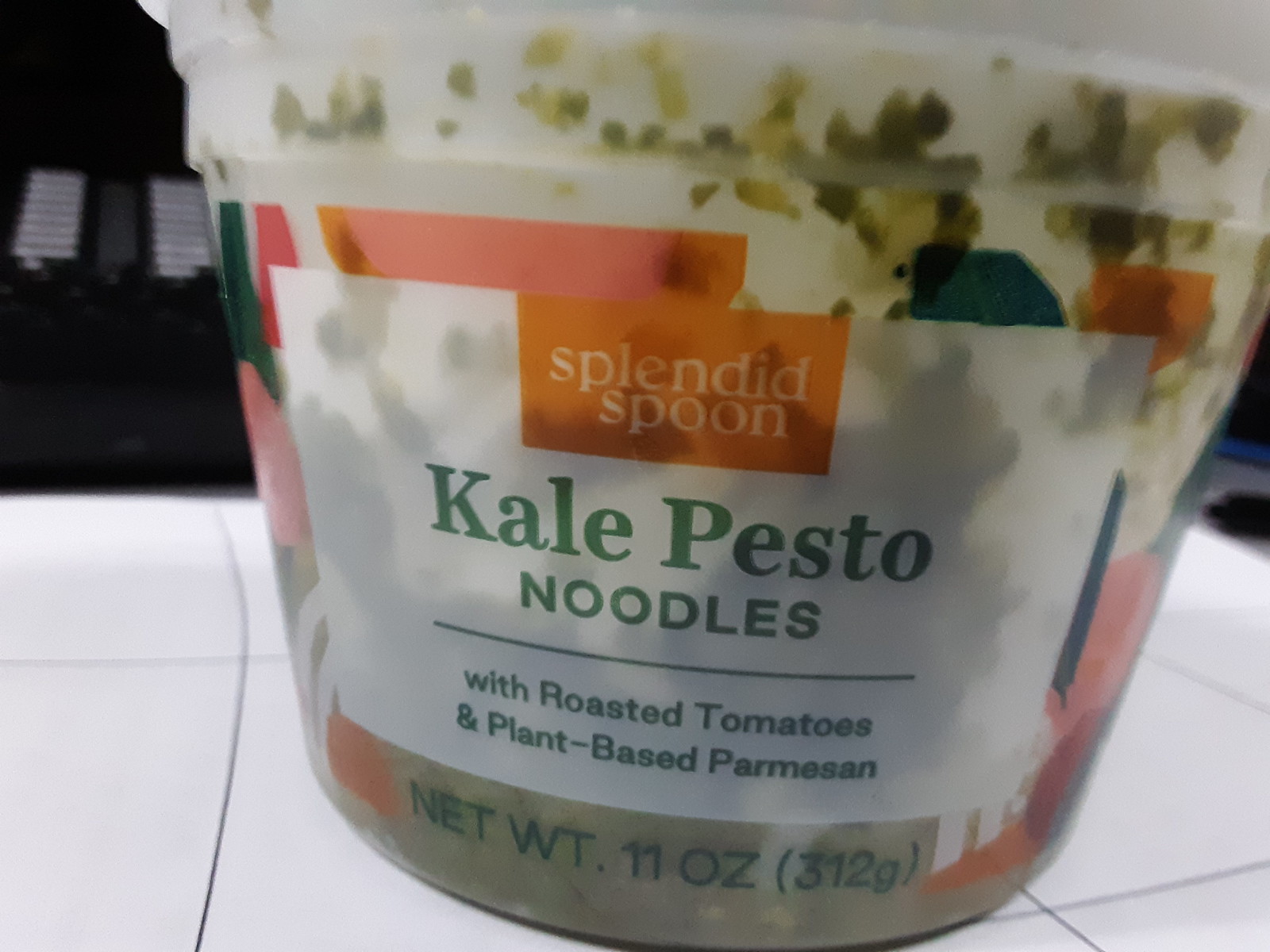This image features a clear, round plastic container of kale pesto noodles from the brand Splendid Spoon. The container is labeled with a large white rectangle in the center edged in an orange border. "Splendid Spoon" is written in light orange within the orange border, while "Kale Pesto Noodles" stands out in large green letters. Below, in smaller green text, it states, "With Roasted Tomatoes and Plant-Based Parmesan." The net weight, "11 ounces (312 grams)," is noted at the bottom of the label in green. The container appears to have been opened and partially consumed, as green specks of pesto and traces of translucent sauce are visible stuck to the inner sides. The package is set on a white-tiled kitchen counter with black grout lines and is positioned against a black wall in the background. The lid of the container is a darker shade of white, adding contrast to the clear plastic body of the container.